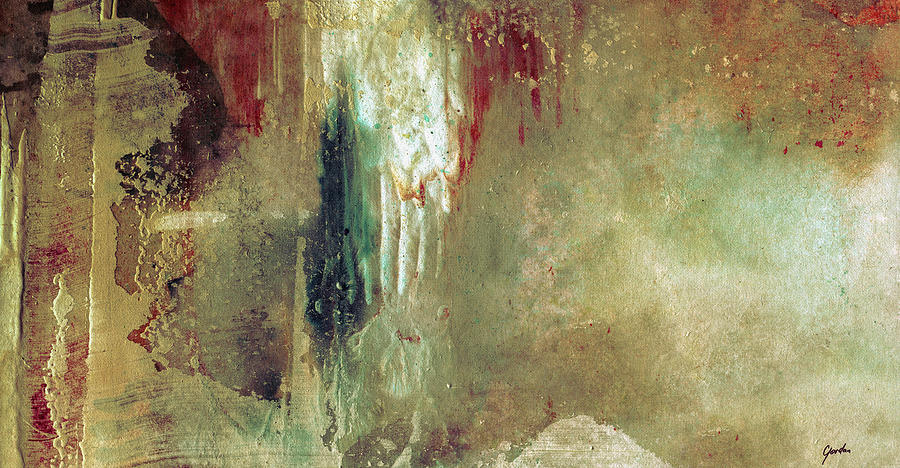A full-color photograph depicts a horizontal rectangular canvas covered in vibrant, abstract art with no border or background, making the painting itself the sole focus. The canvas is an eclectic blend of colors including white, gray, tan, various browns, rich teal green, yellows like mustard, various reds including cranberry and light red, slight purple, and different shades of blue and black. The colors are applied in a chaotic manner, with splatters, smears, dribbles, and speckles, creating a visually stimulating mixture of vertical, horizontal, and circular shapes. Some areas are densely concentrated with paint while others are sparse. In the lower right-hand corner, there's an illegible cursive signature, possibly "Gordon." This piece exemplifies the essence of modern abstract art, where the interpretation is left to the viewer's imagination.